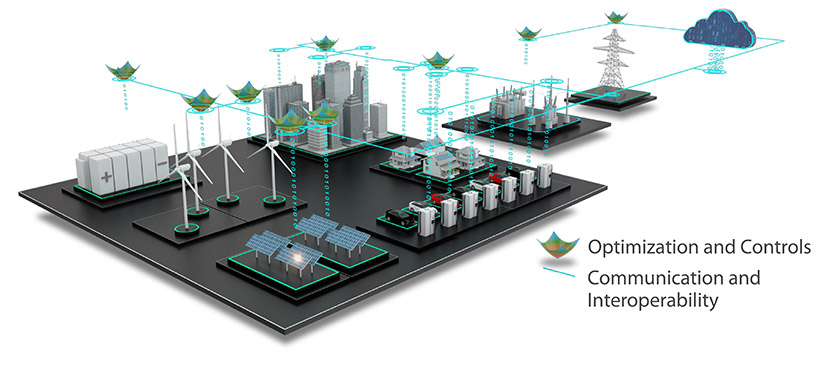The image is a detailed diagram that represents a comprehensive renewable energy system involving solar and wind power. The diagram illustrates various interconnected components of an electrical generator system including solar panels, wind turbines, batteries, electric cars, and a city infrastructure. The solar panels, located in the bottom left of the diagram, are outlined in green with blue or grayish surfaces. Batteries displaying positive and negative signs are scattered on the left and right sides, and there's a charging station for electric cars, which are shown in black, white, and red. 

The top right section of the image depicts a city area with gray buildings. Lines and dotted paths in green and blue denote the communication and interoperability between different sections of the system. A legend to the right annotates these elements, with green lines representing "optimization and controls" and blue lines representing "communication and interoperability." Additional features include a silver tower, a cloud with blue rain, and various electrical items placed on a black platform.

The entire layout appears on a flat blackboard-like surface with the caption "Optimization and Controls Communication and Interoperability" prominently displayed at the bottom right corner in black text on a white background.